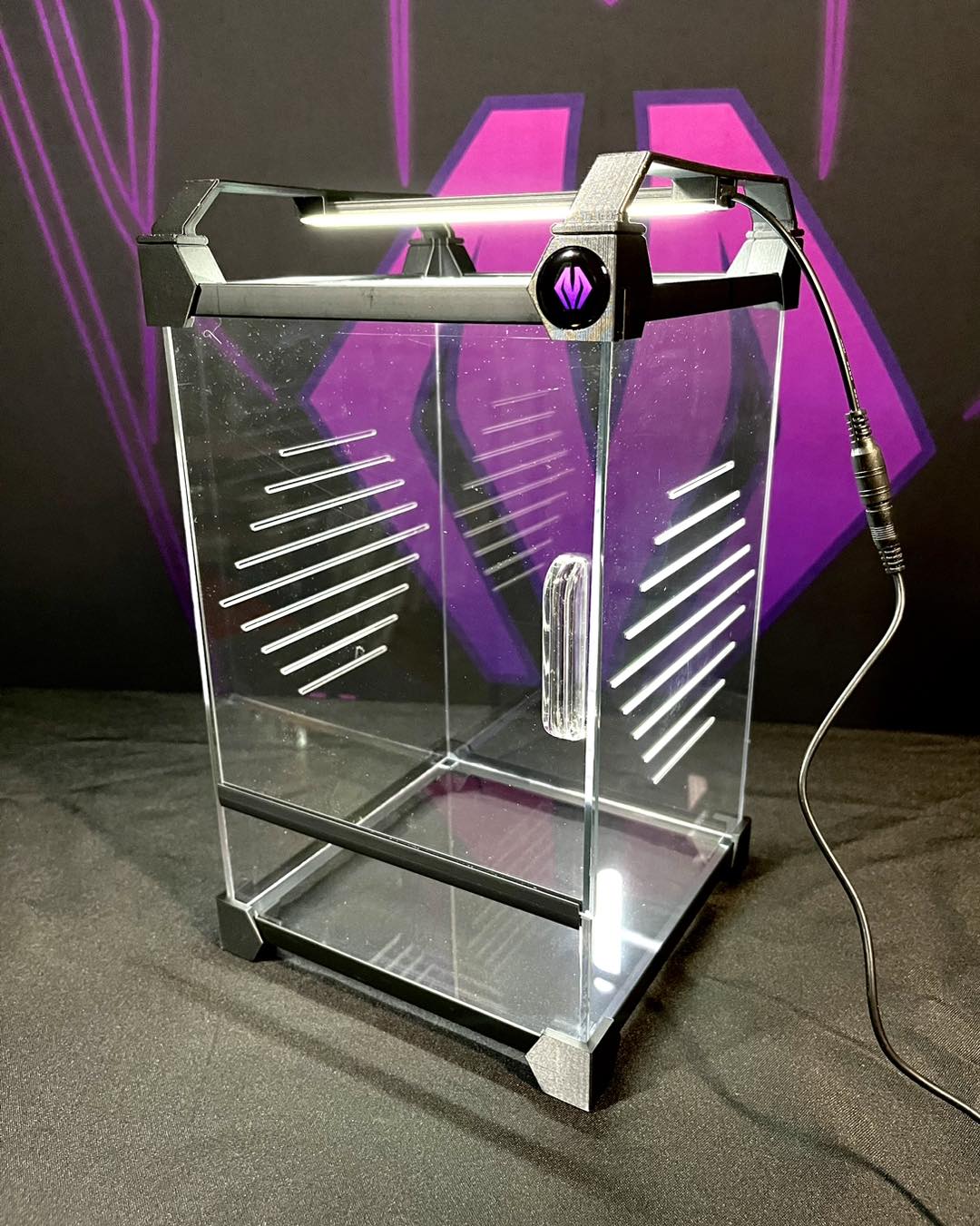The image showcases an empty, tall rectangular box resembling a terrarium or display case, crafted from clear plexiglass or acrylic. The structure stands upright, framed in black, resembling an aquarium design. The box is significantly taller than it is wide, with a square base and a height of at least twice its width. The front features a clear handle used to open a door, while the sides have slats potentially meant for inserting shelving. At the top, a black plastic section houses a fluorescent or LED light strip, with a black cord trailing off to the right. The box rests on a black surface, and the background is predominantly black with purplish-pink markings, including a stylized diamond-shaped "M" logo. The logo on the backdrop matches another similar logo located on the upper right-hand corner of the acrylic box.